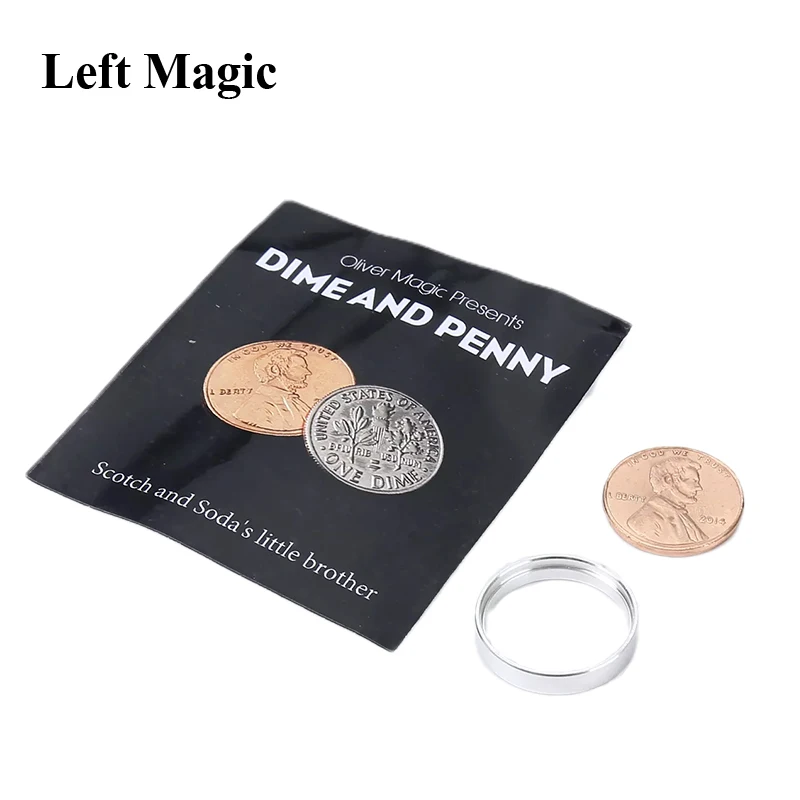The image showcases a product photo of a magic trick set against a white background. The primary focus is a tilted black package in the center, which bears the text "Oliver Magic Presents Dime and Penny, Scotch and Soda's Little Brother." A photograph of a penny and a dime is displayed in the middle of this package. In the top left corner of the image, the words "Left Magic" are prominently displayed. Beside the package on the right, there is an actual penny and a silver ring, both set against a transparent background. The silver ring resembles the size and color of a dime but appears slightly too wide to fit a dime perfectly. The kit seems to include a false back for the penny, hinting at a clever sleight-of-hand trick, potentially involving the illusion of the penny and dime interacting in a mysterious way. The package itself has a slightly wavy appearance, and there is a subtle hint of dust visible on its surface, adding a touch of realism to the promotion.